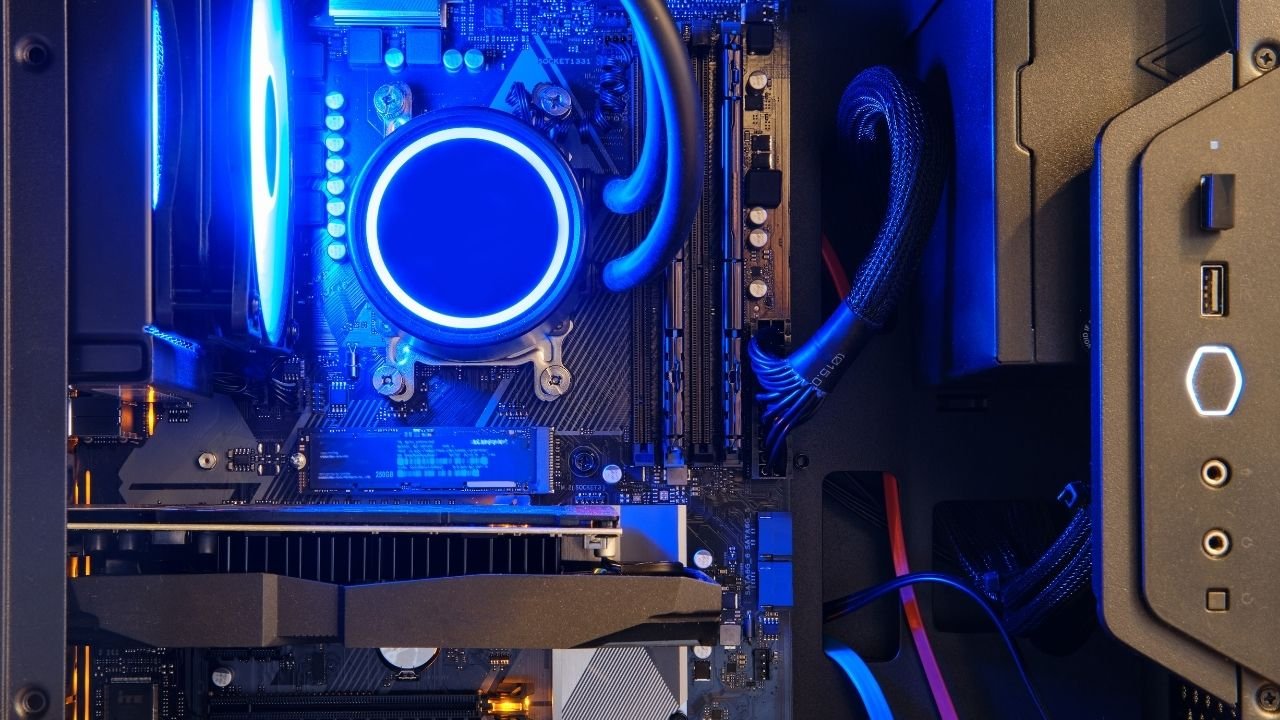The image shows the interior of a computer tower or server, viewed in landscape orientation. The structure is marked by various technical components spread across a rectangular frame of roughly six inches wide and three inches high. On the right-hand side, a raised black panel houses multiple ports, including slots for USB, phone jacks, and headphone jacks. There is also a power button. Adjacent to this panel is a gray, metallic area, possibly part of a power supply unit, and beneath that lies a bundle of thick cables, consisting of red and blue wires, extending towards the left.

Central to the image is a prominent, large circular component, featuring a white center surrounded by a blue neon ring. This element is secured by four screws and is positioned near the top of the structure, emitting a bright, white light. Nearby, bundled wires, possibly power cables, extend towards this circular part, enhancing the technologically dense layout. Below this area sits another gray panel speckled with tiny black holes, just above which additional ports and possibly ventilation fans are seen. A notable point includes several motherboards visible throughout the setup, contributing to the intricate web of electronic components. These various elements underscore the highly detailed and complex nature of the internal workings of the device.